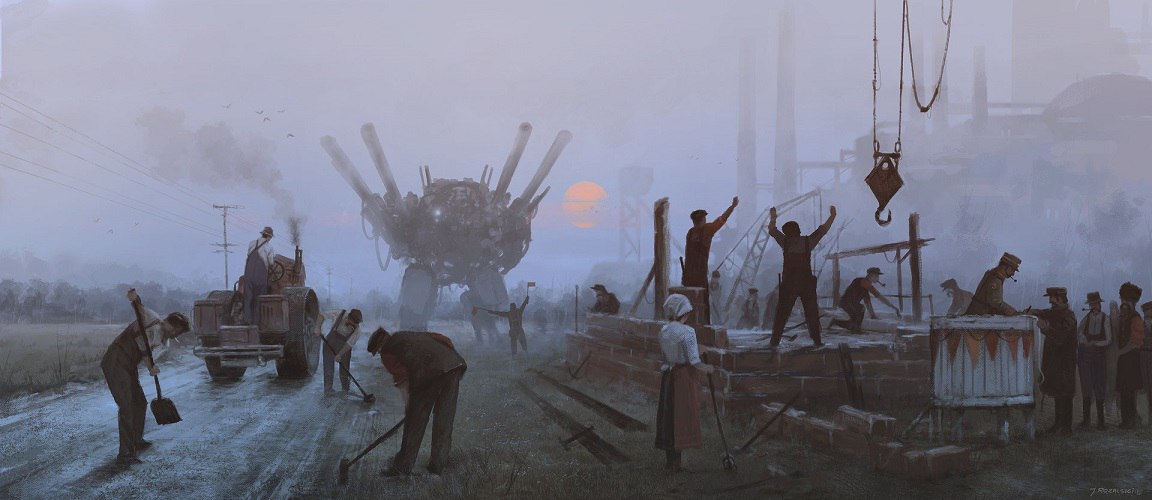The image depicts a post-apocalyptic, steampunk-inspired scene set in an alternative Industrial Revolution era. The painting, characterized by its muted colors of greys and subdued blues, presents a grim and polluted environment. On the right side of the image, a large factory looms, spewing smog into the air. Central to the composition, the Sun, shrouded in haze, is captured either rising or setting. The scene is bustling with activity: in the foreground, men with shovels are engaged in roadwork, while others are busy laying bricks, possibly constructing a building. A person operates a two-wheel tractor nearby. Notably, there is a group of individuals surrounding a man in a hat, seemingly paying him for some service. Dominating the distance, a colossal, menacing piece of machinery, possibly a mech or tank, towers over the workers. One individual appears to be guiding this futuristic vehicle safely through the smog-laden landscape.